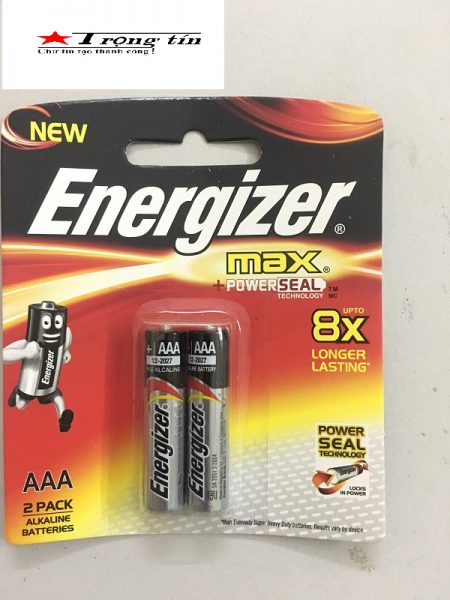The image displays a package of two AAA batteries labeled as "Energizer Max." The design of the packaging appears strikingly similar to genuine Energizer products, featuring vivid colors and light effects typical of the brand. It showcases a gradient color scheme that transitions from black at the top to gray at the bottom right, with striking accents of red and yellow in the middle. A notable deviation from authentic packaging is the inclusion of a low-quality battery mascot that is not the recognizable Energizer Bunny. Additionally, in the top left corner, there is a label with the text "Trong Tin," which may indicate Vietnamese origins or influence, although it is unclear if this detail was digitally added to the picture. The package proclaims "Energizer Max plus power seal technology" and claims to offer up to eight times longer battery life. Despite its efforts to mimic official Energizer branding, certain elements suggest that this product might be a knock-off.